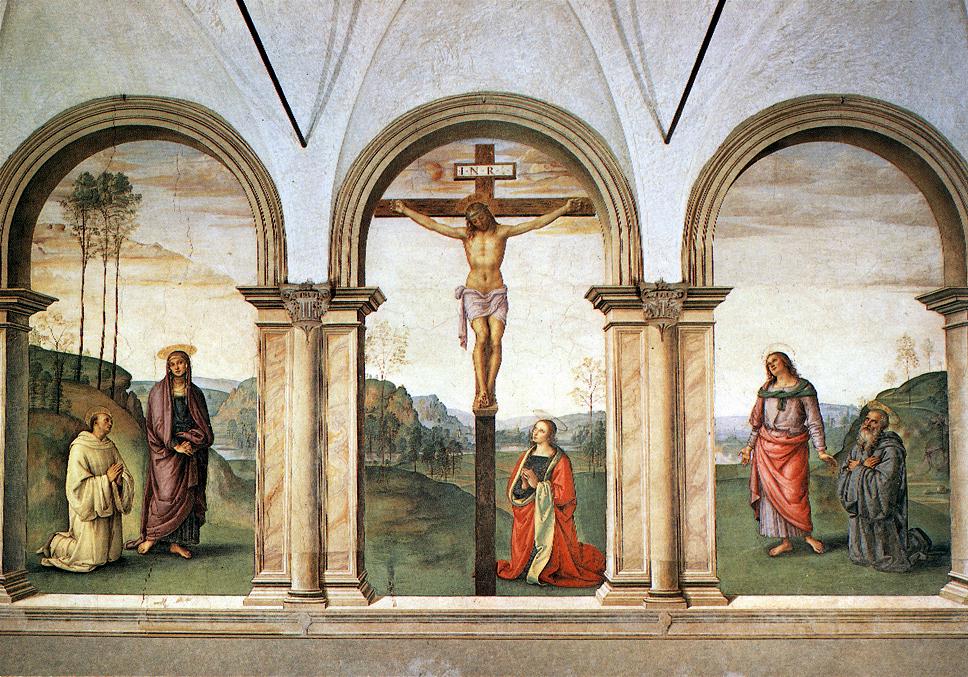This vividly detailed painting depicts the crucifixion of Jesus Christ and is characterized by its rich colors and intricate elements. At the center, Jesus is shown on a tall, brown cross, crowned with thorns and with nails piercing his hands and feet. Above his head is the inscription "INRI." Surrounding the cross are five figures, all with halos, signifying their sanctity. Directly beneath Jesus, Mary Magdalene, identifiable by her red robe, is on her knees in prayer. To the left, a kneeling monk-like figure also prays, accompanied by a standing woman. On the right, a man kneels in supplication, while a woman stands beside him, gazing at Jesus. The background reveals an elaborate setting with structured stone pillars, arches that may signify a church, and a vibrant garden. The colors green, white, red, black, and purple enrich the scene, adding depth and dimension to this masterfully crafted depiction of a religious moment.